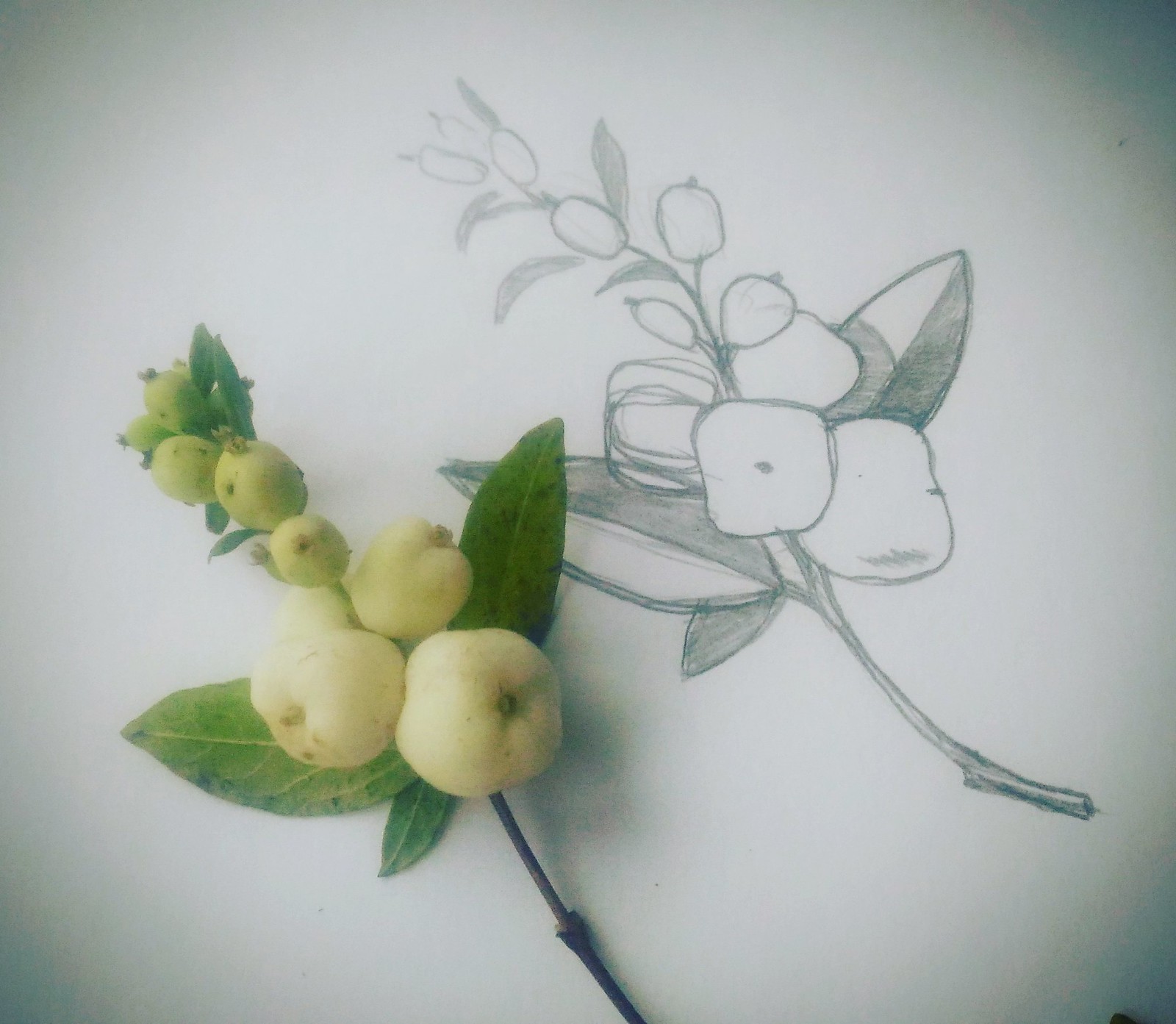In this rectangular image, we are presented with a top-down view of a photograph showcasing both a pencil sketch and the real-life subject it depicts. Starting from the lower left corner, a realistic plant branch is visible, featuring a slender stem and small fruit that resemble miniature pears. This branch extends diagonally from the center-bottom toward the upper-left corner. The fruit, a pale green color, tapers from a plump base to a narrower top and is surrounded by almond-shaped green leaves.

Positioned to the right of the actual plant branch is a pencil sketch attempting to capture the same subject. The sketch shows the branch and fruit, though the artist appears to be somewhat inexperienced. The shading on the leaves is not expertly done, and the representation of the fruit lacks detailed shading, indicating a novice effort. Nevertheless, it’s clear that the artist’s intention was to recreate the plant branch as accurately as possible.